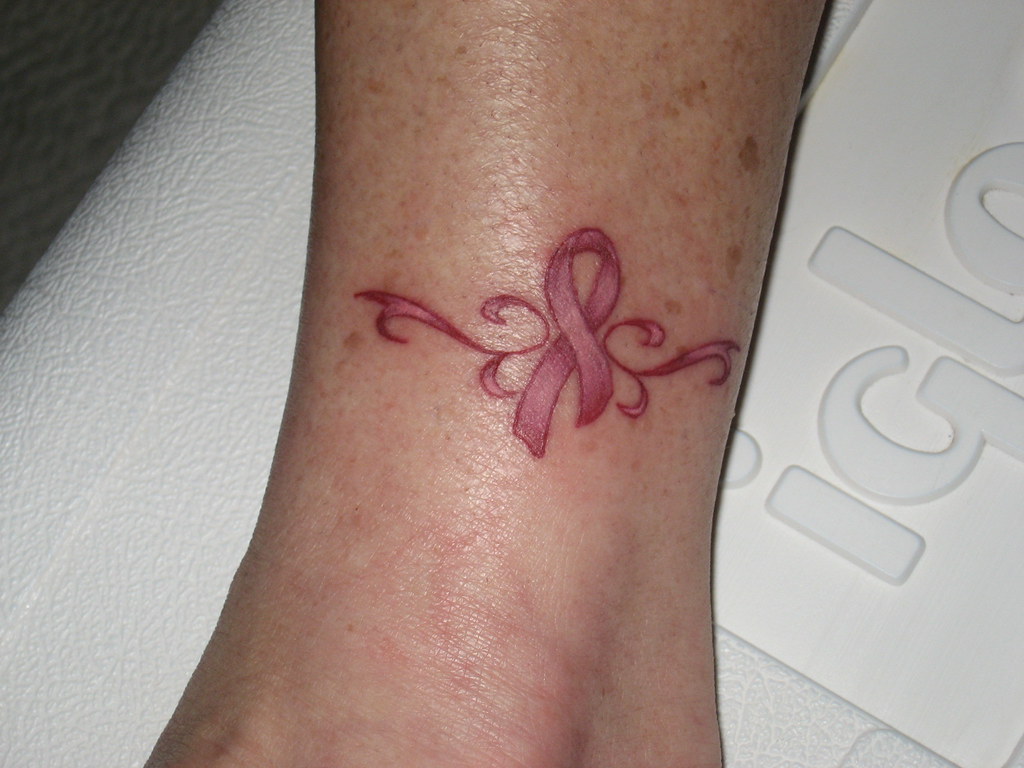This close-up photograph captures a white, thin ankle resting atop the white lid of an Igloo cooler, with the cooler's logo, "IGLOO," visible on the right side. The focal point of the image is a recently inked tattoo located on either the person's ankle or wrist. This tattoo features a pink or red bow at its center, which resembles a Hallmark symbol or possibly a cancer awareness ribbon, and is adorned with artistic filigree designs extending from each side. The skin around the tattoo is slightly irritated, indicating it is fresh. The ankle and limb, presumed to be that of a woman, display numerous age spots and moles, suggestive of significant sun exposure over time. In the background, a white area and a dark green section can be observed, adding contrast to the detailed image.